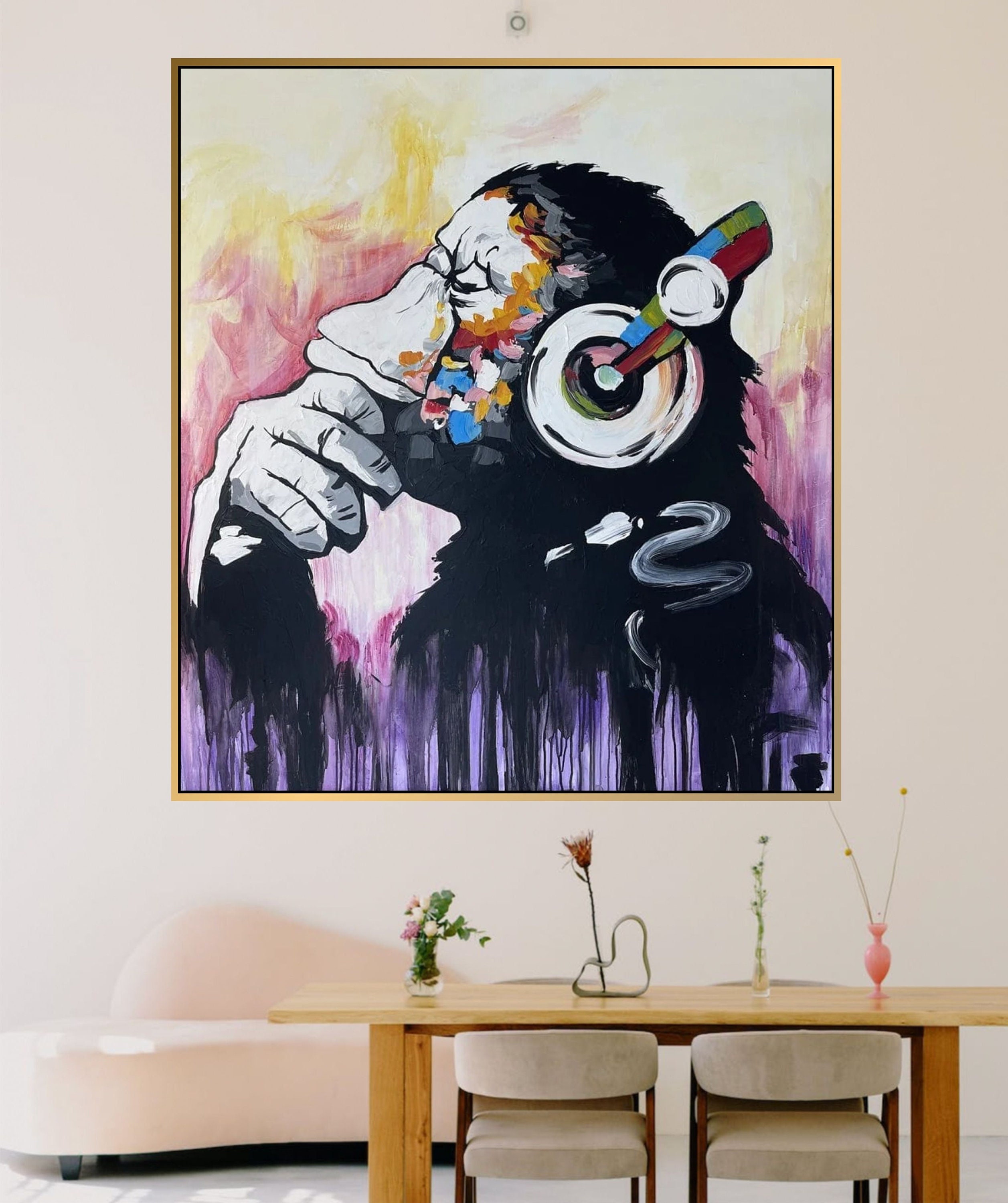The photograph captures a stylish and meticulously arranged room, blending elements of a dining and living area. Central in the foreground stands a modern wooden table with brownish wooden legs and a blond wood top. The table features a collection of four eclectic sculptures arranged from left to right. The first is a small vase with flowers and greenery; next is a metallic sculpture resembling a long flower; then, a glass rod sculpture adorned with green dots; and finally, a pink vase with two long, antenna-like protrusions. Two chairs with white cushions and backs are placed on either side of the table.

Behind the table sits a light pink, curved modern sofa positioned against a pristine white wall. The photograph's focal point is a captivating painting mounted on the wall in a slender gold frame. This artwork features a left-profile of a contemplative chimpanzee, vividly portrayed with its right hand resting beneath its chin. The chimp's face is predominantly white, contrasting with its dark, purple-streaked fur. It sports colorful cylindrical headphones with a combination of blue, green, and red on the band and silver over the ears. The face is accentuated with whimsical whiskers and vibrant color patches in blue, red, white, and green.

The background of the painting is a symphony of colors, predominated by purple and magenta hues with yellow highlights, set against a greenish-beige tone. Above the painting, a small white camera is subtly installed, adding a layer of modern surveillance or monitoring to the scene. The room's arrangement, coupled with the striking artwork, suggests a blend of modern aesthetic with playful artistic elements, creating a visually engaging and thought-provoking space.